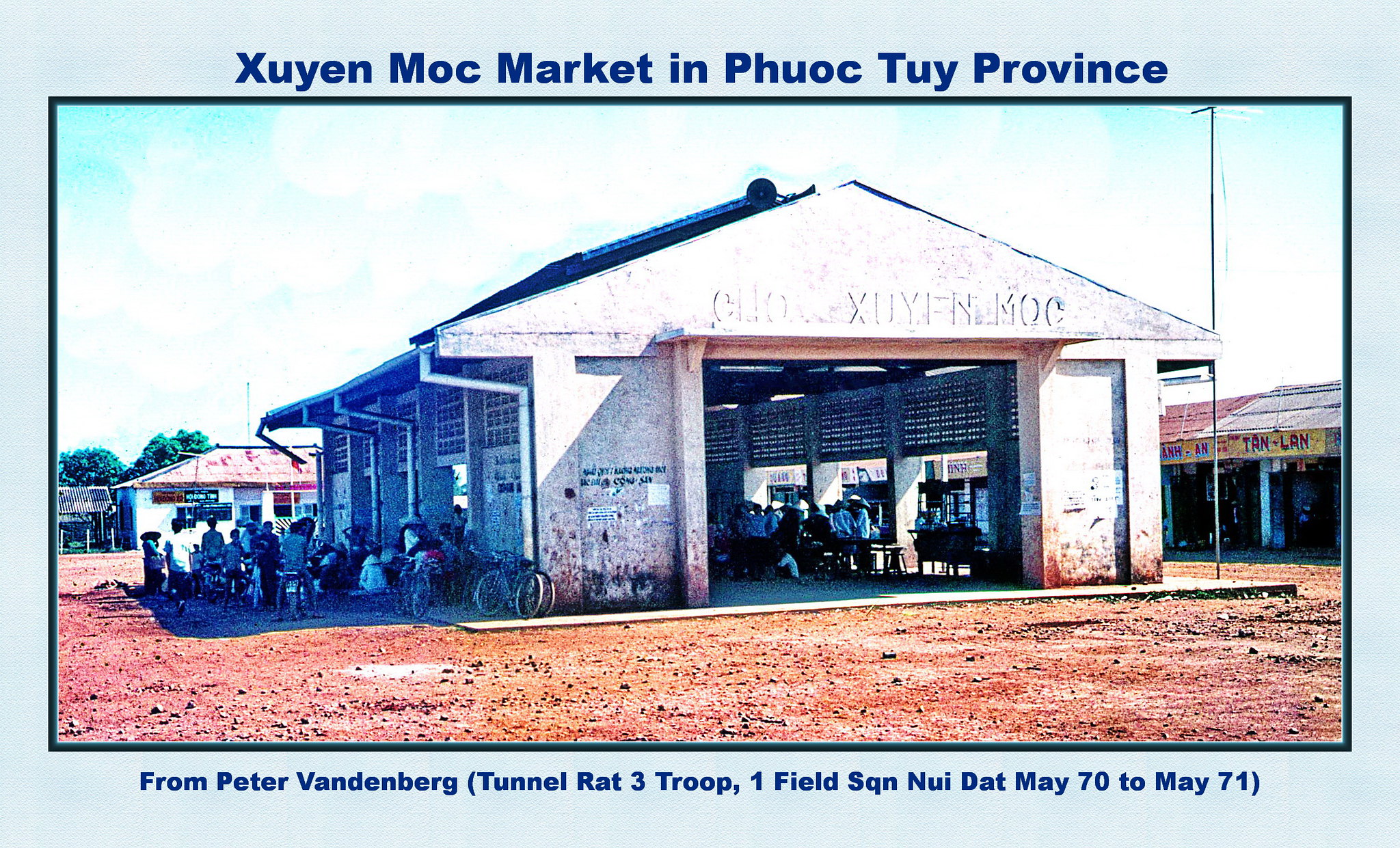This photograph captures the lively scene of the Xuyen Moc Market in Phuoc Thuy province, Vietnam, documented by Peter Vandenberg of Tunnel Rat Troop 1, Field SQN Nui, from May 1970 to May 1971. The central focus is a two-story cement building with a triangular top, marked by the faint text "Xuyen Moc" on its facade. The building features an open garage-like entrance, allowing people to freely enter and exit, and is situated at a corner.

Inside, the building seems to serve multiple purposes: there's a motorcycle shop area with bikes parked in the left quadrant, and possibly a cafe with tables where people are seated, suggesting a communal space. The sky above the building is overexposed and blown out, creating a stark white backdrop. Along the side of the building, numerous bicycles are parked against the wall, and various people are visible, contributing to the bustling market atmosphere. The contrast between the brown soil in the foreground and the beige color of the building accentuates the vivid life and structure of this corner market. A shorter building can be seen on the right edge of the image, adding to the layered complexity of the scene.